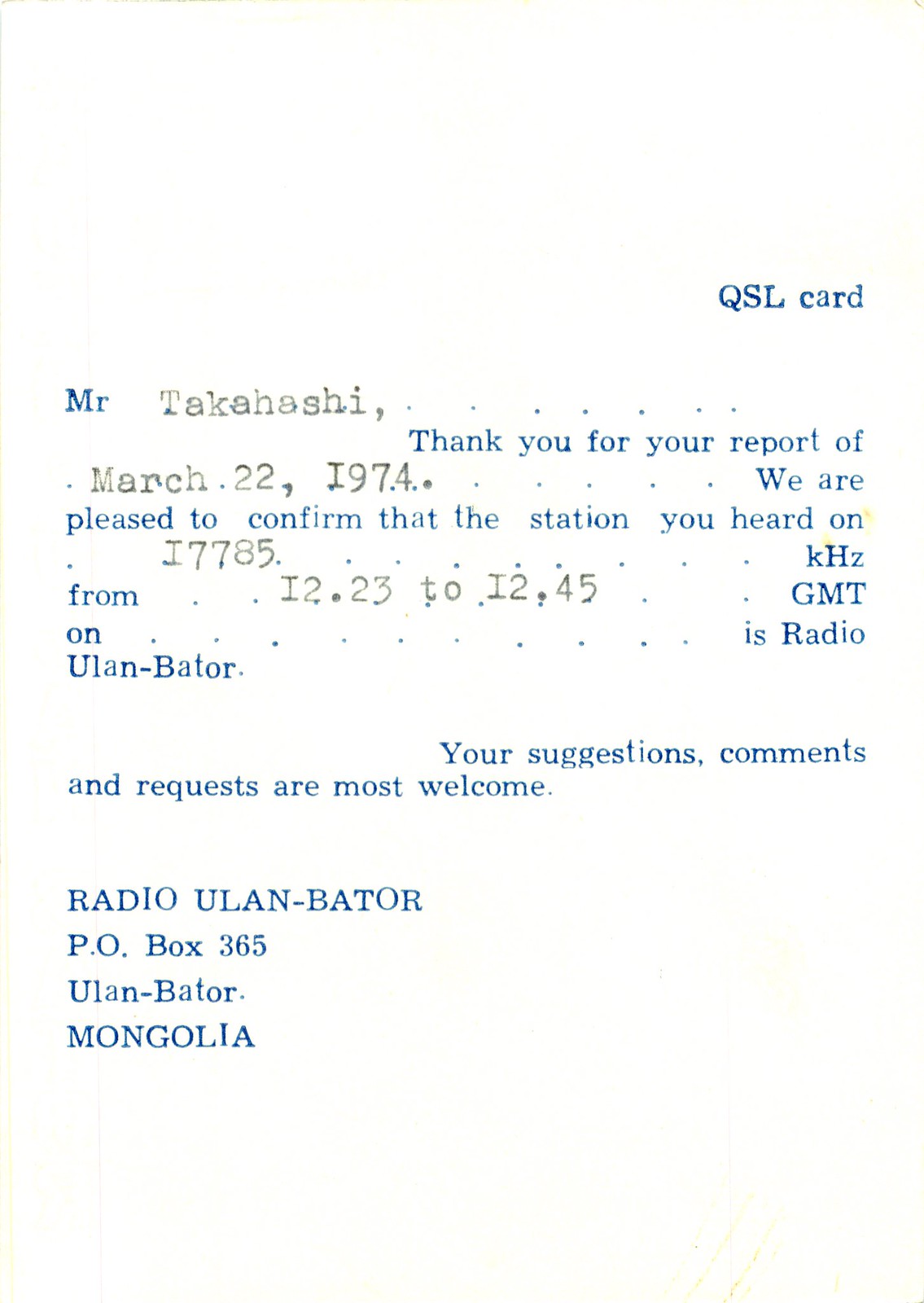The image features a white piece of paper with a combination of blue and black text. At the top, it prominently says "QSL card" in blue. Following this, the salutation "Mr. Takahashi" combines blue "Mr." and black "Takahashi." The letter continues in blue: "Thank you for your report of," followed by the date in black: "March 22nd, 1974." The confirmation text in blue reads, "We are pleased to confirm that the station you heard on," and in black: "17785 kHz" from black: "12.23 to 12.45 GMT." The closing part in blue states, "Your suggestions, comments, and requests are most welcome." At the bottom, in blue, it says: "Radio Ulaanbaatar, P.O. Box 365, Ulaanbaatar, Mongolia."